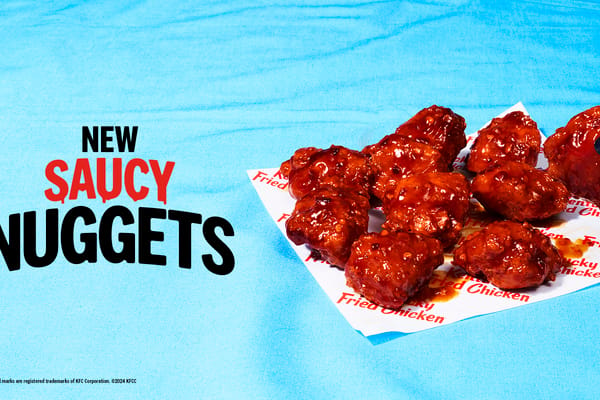The image features a vibrant advertisement for new saucy nuggets. On a bluish, lightly waved background that resembles blurred fabric, bold text is prominent on the left. The text consists of three rows: "New Saucy Nuggets." The word "Saucy" is in dripping red letters, while "New" and "Nuggets" are in bold black, with the "N" in "Nuggets" partially cut off on the left side. 

To the right of this text, there is a white napkin patterned with the words "Kentucky Fried Chicken" in red, placed diagonally. Positioned casually on top are glistening saucy nuggets, reddish-orange in color with a textured, round, and slightly irregular shape. The sauce, rich and vibrant, appears to contain bits of peppers, adding to the enticing visual appeal, and some of it is smeared on the napkin. The nuggets' succulent, saucy appearance contrasts appealingly with the clean blue background and the crisp white napkin beneath them.